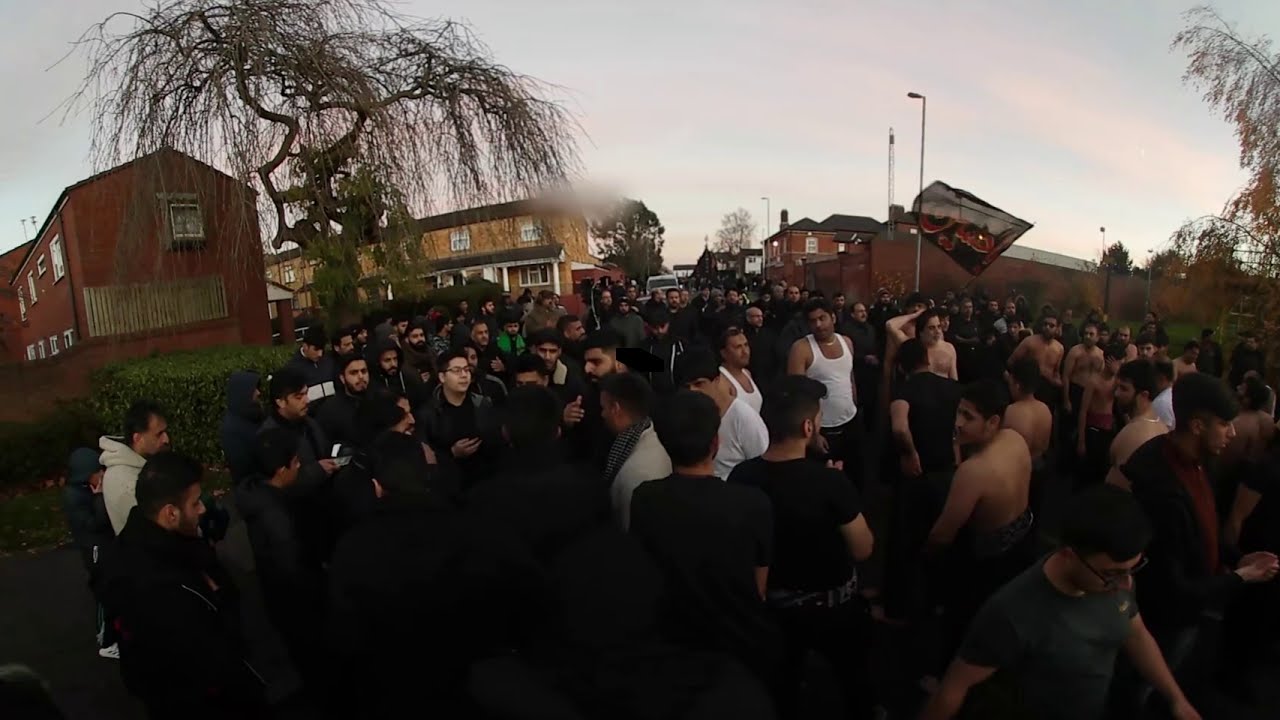The image depicts a large gathering of young men, predominantly wearing black or gray clothing, with a few in white tank tops or shirtless. They have uniformly short, dark hair and are clustered tightly on a street in a residential area, appearing engaged in conversation or looking at one another. In the background stand two-story brick apartment buildings, primarily in shades of brown, yellow, and red. The crowd is so dense that it stretches across the entire width of the image and extends into the distance. Above the crowd on the right side of the image, a black flag with red Arabic text is visible. Trees, some barren, and hedges are scattered along the top and sides of the photo, contributing to a hazy sky that illuminates the scene with a muted brightness. The overall setting might be a public housing estate or potentially near a park.